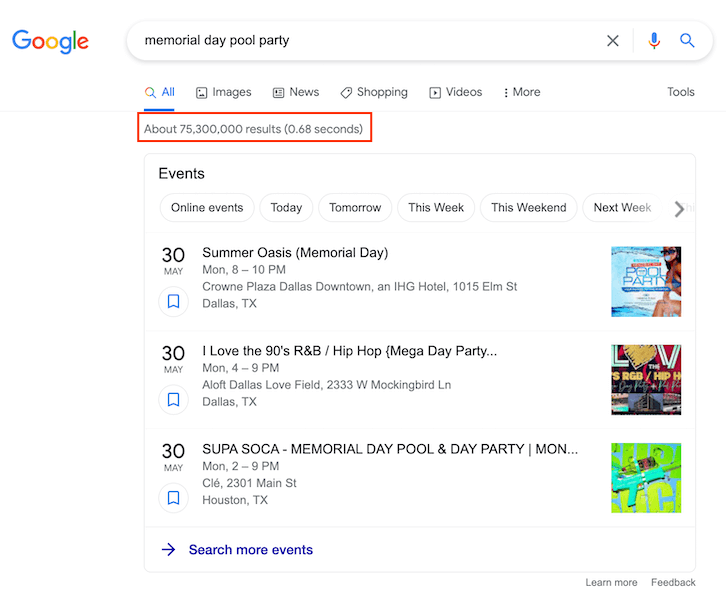The screenshot captures a Google search page on a desktop computer. In the top-left corner, the colorful Google logo is prominently displayed: a blue 'G', a red 'O', a yellow 'O', a blue lowercase 'g', a green 'l', and an orange 'e'. To the right of the logo, the search query "Memorial Day Pool Party" is entered in the search bar. Below the search bar, there are several categories: All (highlighted in blue), Images, News, Shopping, and Videos. A red outline emphasizes the search result count, which is approximately 75,300,000 results found in 0.68 seconds.

Directly beneath this, under the heading "Events," options for online events span today, tomorrow, this week, this weekend, next week. The first listed event is the Summer Oasis Memorial Day event on May 30th, scheduled from 8 to 10 PM at the Crowne Plaza in downtown Dallas (1015 Elm Street, Dallas, Texas). Another event on May 30th is the "I Love the 90s R&B/Hip-Hop Mega Day Party," running from 4 to 9 PM at Aloft Dallas Love Field, also in Dallas, Texas. Finally, the Supa Soca Memorial Day Pool and Day Party is scheduled for May 30th, from 2 to 9 PM in Houston, Texas.